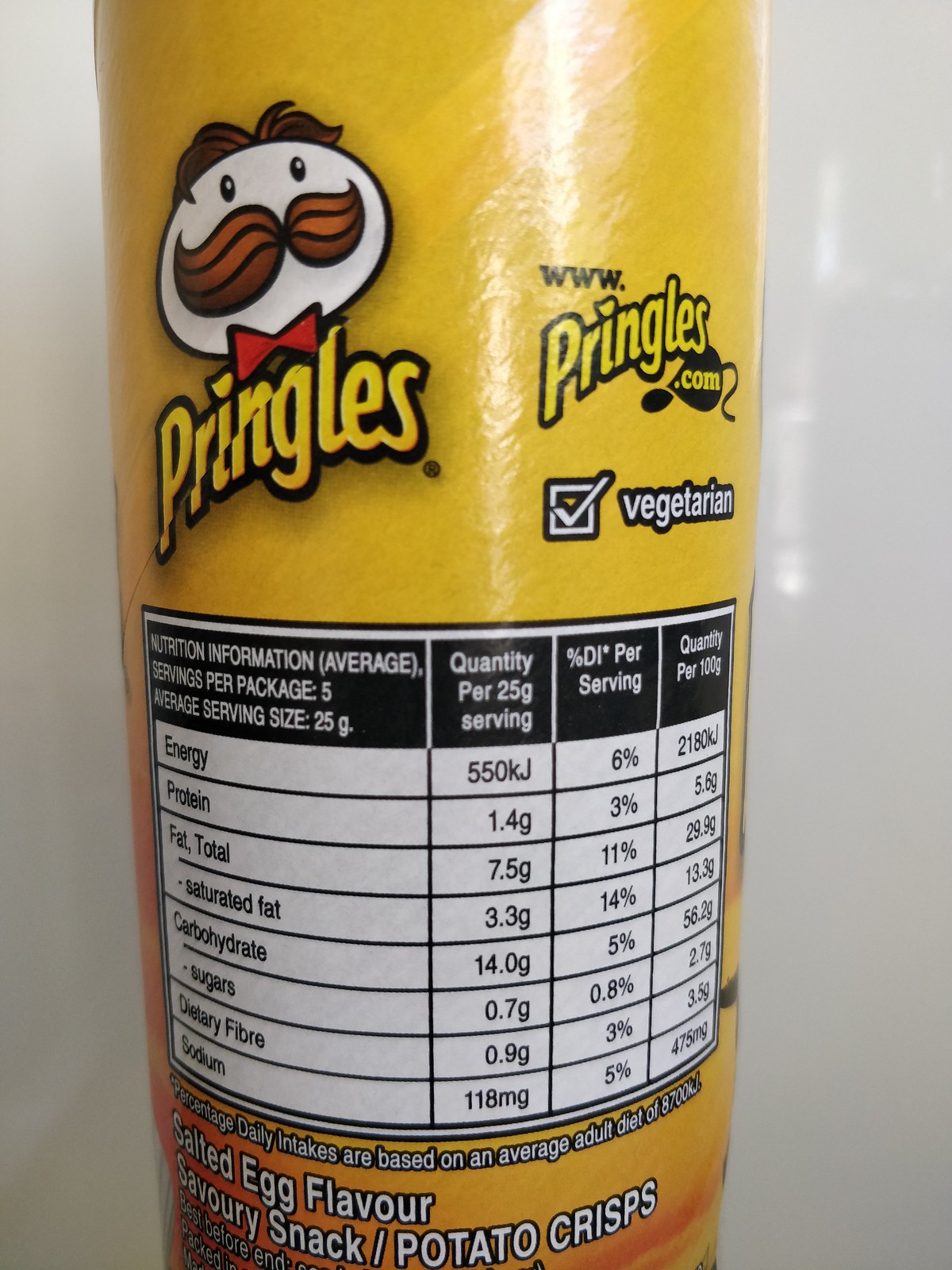The image showcases a bright yellow cylindrical can of Pringles against a white background. Prominently displayed on the upper left is the iconic Pringles logo, featuring a stylized man with a brown mustache, tuft of black hair, beady black eyes, and a red bow tie, along with the yellow text "Pringles." To the right of the logo, the text "www.pringles.com" is shown in black and yellow next to a white square with a checkmark and the word "Vegetarian." The center of the can features a large, white, black-labeled nutritional information chart detailing average servings per package (5), average serving size (25g), and nutritional values such as energy, protein, total fat, saturated fat, carbohydrates, sugars, dietary fiber, and sodium. Below this chart, white text provides additional product details, including "% Daily Intakes are Based on an Average Adult Diet," "Salted Egg Flavor," "Savory Snack," and "Potato Crisps." The glossy finish of the packaging reflects light, emphasizing its shiny surface.